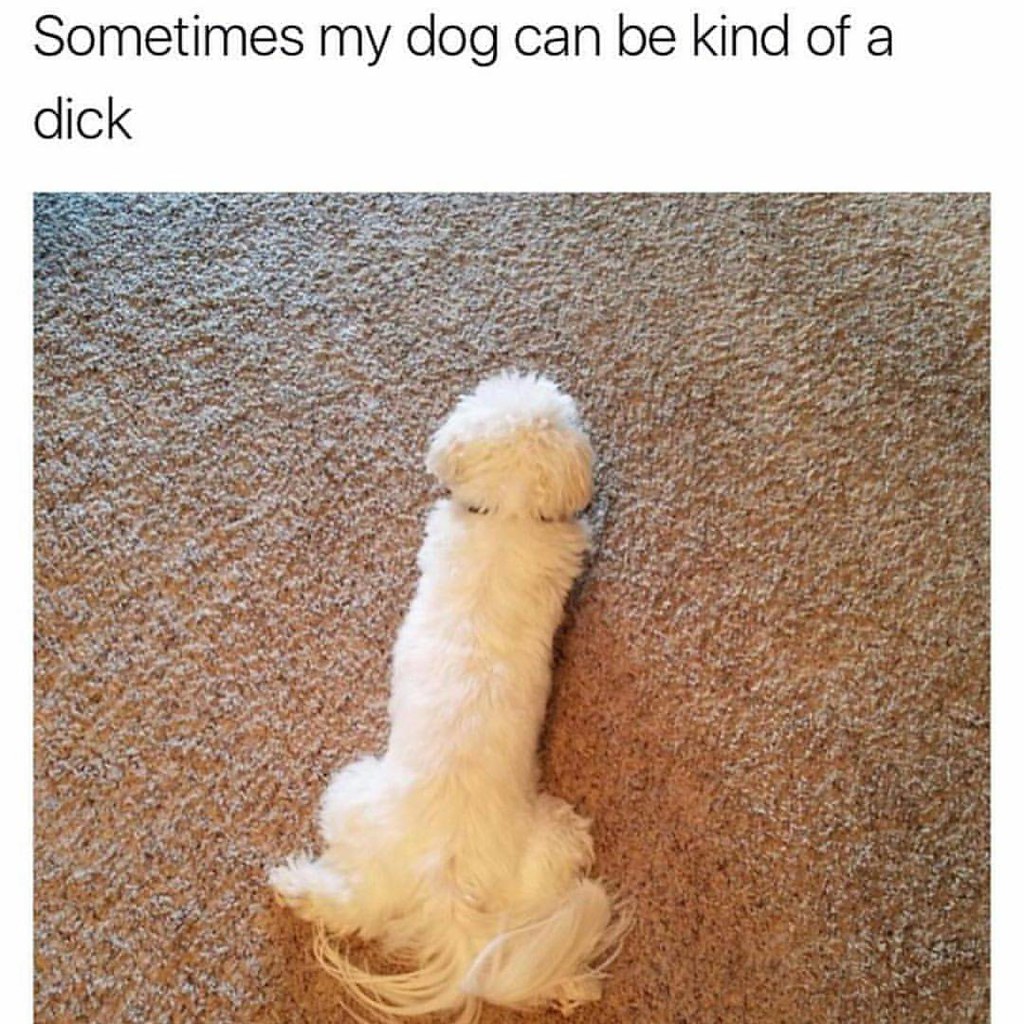This image features a bright white, fluffy Shih Tzu-like dog laying on a short, fuzzy, brown carpet inside a room. The photo, taken from above, humorously resembles a phallic shape, with the dog’s body contoured in a way that its back legs are stretched out, its belly against the carpet, and its tail with long strands of hair trailing behind. The dog wears a brownish collar around its neck. Overlaying the image on a white background, a caption in black lettering reads, “sometimes my dog can be kind of a D-I-C-K,” making a playful reference to the humorous shape. The overall effect is intended as a meme, joking about the dog's position and appearance.